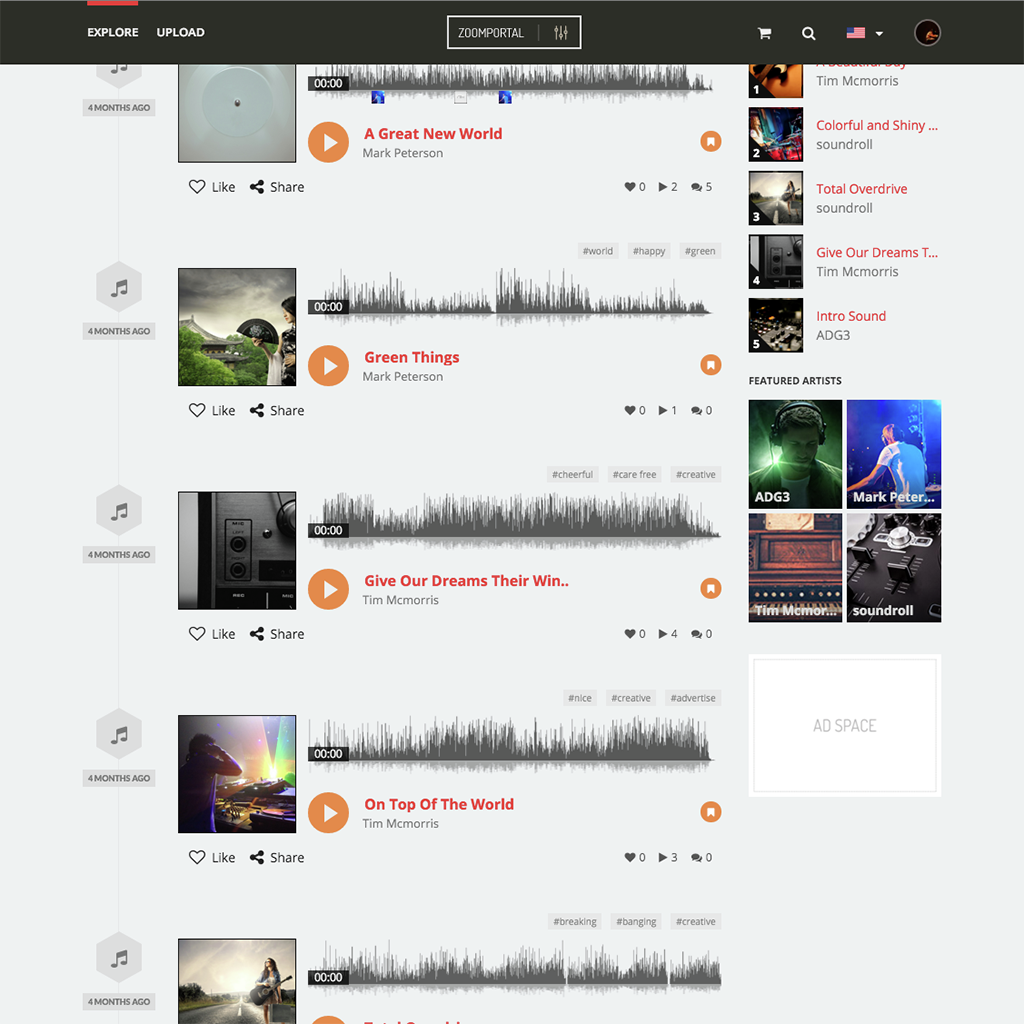This image is a screenshot of a music website with a structured and detailed layout.

At the top of the screen, there is a black header spanning the top inch of the page. On the left side of this header, about an inch from the edge, the word "EXPLORE" is displayed in bold, white, capital letters. Directly above "EXPLORE," a thin red bar is visible. To the right of "EXPLORE," a white "UPLOAD" button occupies the center of the header.

Below the header, a prominent black rectangle with a white border catches the eye. Inside this rectangle, "ZOOM PORTAL" is written in all capital, white letters. Adjacent to this text, a small gray line separates it from three vertical gray lines with a gray circle placed on top, bottom, and middle.

Towards the far right, about an inch from the edge, there is a black circle with a gray border. To its right, an upside-down white triangle sits alongside an American flag, a white search icon, and a white shopping cart icon. The background beneath these elements is a light blue color.

On the left side of the page, there are five small square boxes stacked vertically, each displaying a music note icon. Below each music note, a time stamp indicating "four months ago" is visible. To the right of these squares, images of album covers are presented. Beneath each album cover, icons for "LIKE" (accompanied by a heart), "SHARE" (accompanied by a share icon), and a sound wave bar stretch horizontally. Below the sound wave bar, an orange circle with a white play button is visible. The song title is written in red, with the artist's name below it in black.

On the right side of the album covers, there are interactive elements: an orange circle with a white bookmark icon, a black heart with a numerical count, a black play button with a numerical count, and a comment button with a numerical count. These elements repeat down the column for all five listed songs.

To the far right of these interactive elements, there are five album cover images. Below each cover, the song title is displayed in red, the artist's name in black, and the featured artists below that. Two additional thumbnail images are found underneath the featured artists.

At the bottom of the screenshot, there is a white square labeled "AD SPACE" in black text.